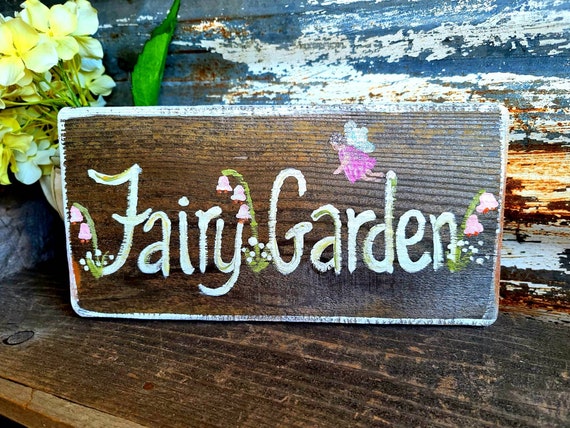This up-close photograph captures a rustic scene with a wooden sign resting on a matching chestnut-colored wooden surface. The backdrop is a weathered, scraped wall featuring tones of blue, white, and hints of brown, adding to the overall vintage aesthetic. On the left side of the image, behind the sign, sits a white ceramic vase with fake hydrangea flowers in a yellow hue.

The sign itself is a stained chestnut wood rectangle adorned with a painted white border. In white, the sign reads "Fairy Garden." Above the word "garden," a small fairy in a pink dress with white wings is depicted. Pink flowers, resembling bluebells or forget-me-nots, are artistically scattered around the text, adding a whimsical touch. The detailed portrayal of the fairy and flowers around the sign creates an enchanting and cohesive fairy garden theme.